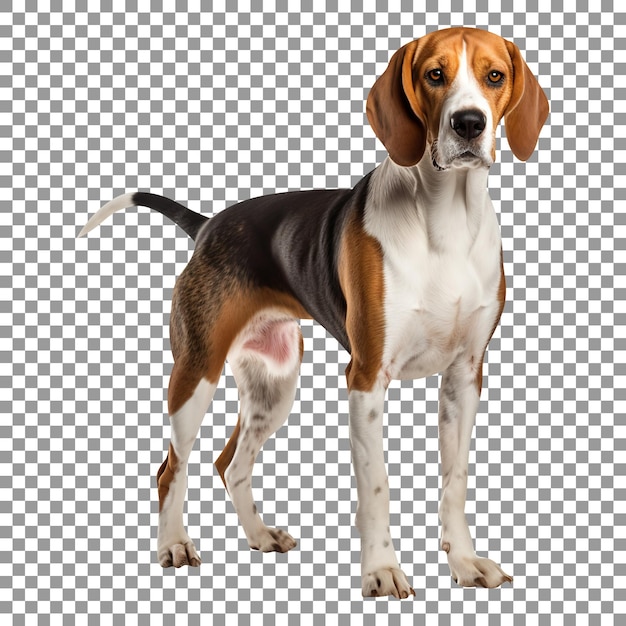The image features a medium-sized beagle dog standing diagonally on a gray and white checkered background, which likely indicates a transparent background. The dog has a predominantly black back with brown highlights on the shoulder and hip joints extending down to the legs. Its legs are mainly white, though the back legs have some brown patches. The dog's face is primarily brown with a white snout and a black nose, and it wears a somewhat sad expression. Its ears are floppy and brown, while its neck and chest are white. The tail is mostly black with the last quarter turning white. The image is square-shaped, and apart from the dog, there are no other components present.